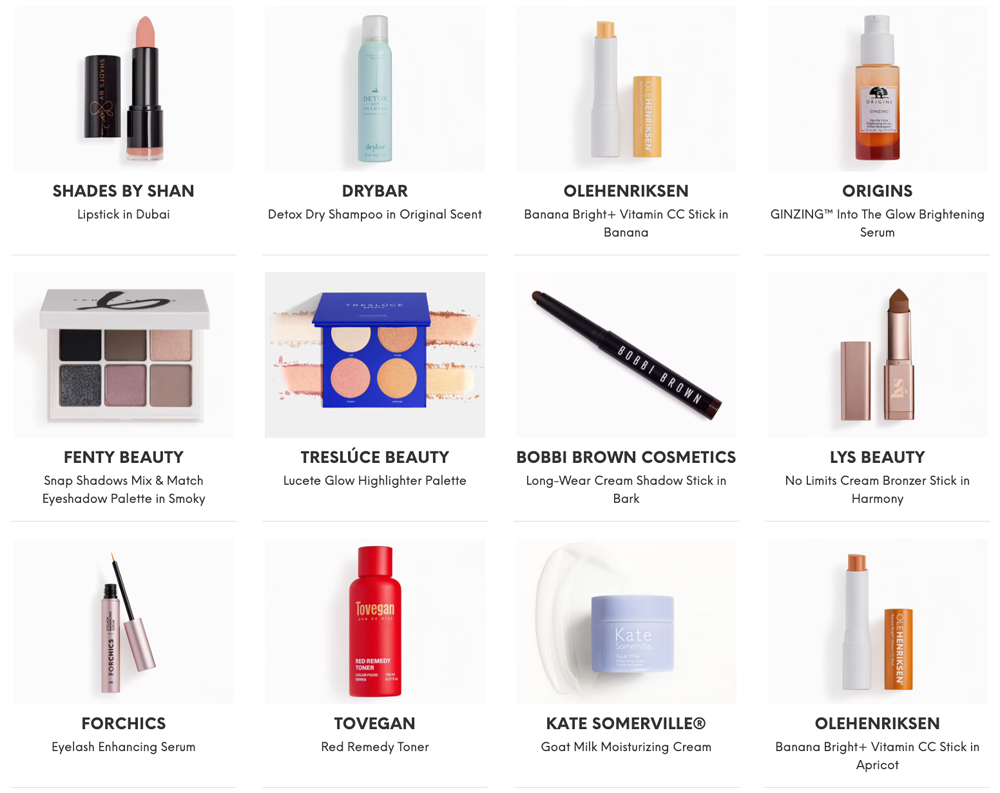A curated collection of diverse beauty and skincare products is showcased. Among the items, there's a "Shades by Shaun Lipstick" in the color Dubai, known for its rich and vibrant hue. The collection also includes "Drybar Detox Dry Shampoo" in its classic Original scent, perfect for refreshing hair between washes. Other notable items are "Ole Henriksen Banana Bright + Vitamin C Serum Stick" and the "Origins GinZing Into the Glow Brightening Serum," both aimed at enhancing skin radiance.

For those looking to create stunning eye looks, the "Fenty Beauty Snap Shadows Mix & Match Eyeshadow Palette" in the Smokey tone provides versatile options. Adding a touch of luminescence, "Trust Fund Beauty's Loose Powder Trust Fund" and the "Blue Creek Glow Highlighter Palette" offer shimmering highlights.

"Bobbi Brown Cosmetics Long-Wear Cream Shadow Stick" in Bark presents a creamy, enduring option for eye makeup. The collection also features the "LYS Beauty No Limits Cream Bronzer Stick" in Harmony, perfect for contouring and adding warmth to the complexion. For lavish lashes, there's the "ForChics Eyelash Enhancing Serum."

Toning and moisturizing essentials are represented by "Tata Harper's Vegan Red Remedy Toner," "Kate Somerville Goat Milk Moisturizing Cream," and another appearance of the "Ole Henriksen Banana Bright + Vitamin C Stick" in Apricot. This array of high-quality products offers a comprehensive selection for beauty enthusiasts.